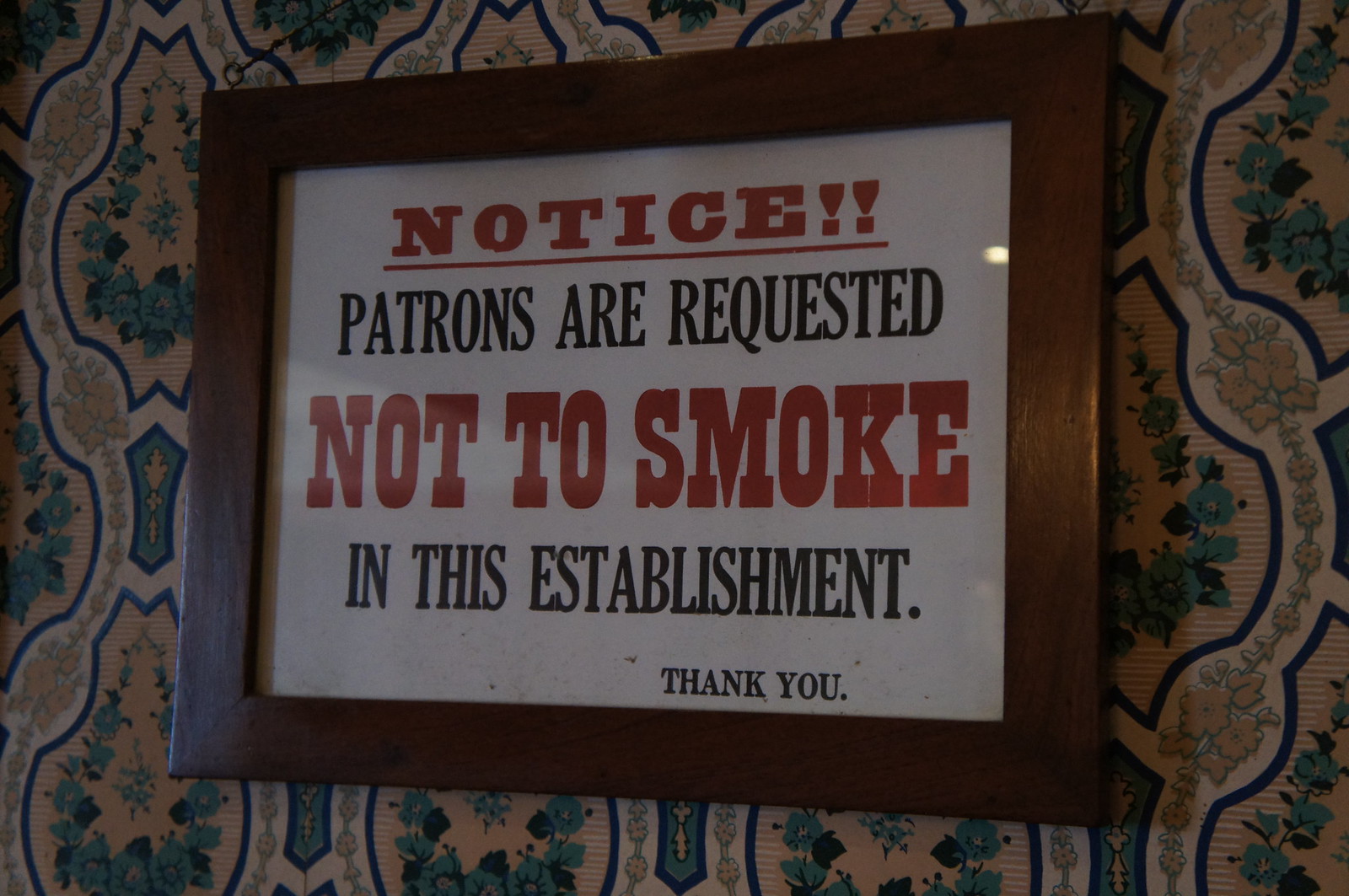The image features a prominently centered sign within a dark brown wooden frame mounted on a wall adorned with vintage-style wallpaper. The sign has a white background and contains a polite request in bold red and black text. The header reads "Notice!!" in large red letters with an underline, followed by the message, "All patrons are requested not to smoke in this establishment." The critical phrase "not to smoke" is emphasized in the largest red font, while the words "in this establishment" and "thank you" are in smaller black text. The wallpaper surrounding the sign showcases a classic floral pattern with muted tones of whites, yellows, greens, blues, and turquoise. The setting likely resembles an indoor space such as a restaurant or bar with dim lighting, contextualizing the sign's directive within a public setting.